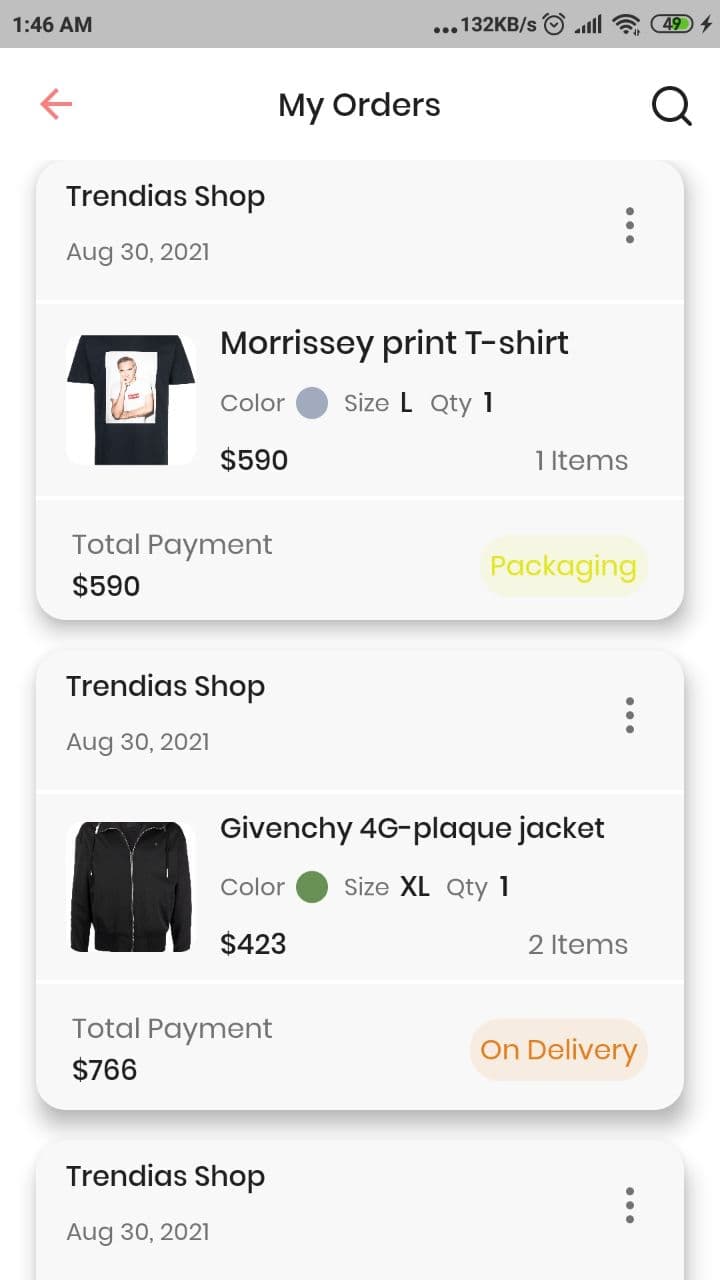A screenshot captured at 1:46 a.m. shows various on-screen indicators: a battery at 49%, internet speed of 132 kbps, a Wi-Fi icon, and an alarm icon. The top section of the screen includes an ellipsis, the title "My Orders," a red arrow pointing left, and a magnifying glass on the right. Below this, a gray rectangular box is labeled "Trendia's Shop, August 30, 2021," with a preview of the first item ordered: a black t-shirt featuring an indistinct person in a central box. The item is described as a "Morrissey Print T-Shirt," color gray, size large, with a quantity of one, priced at $590, and the "Total Payment" listed as $590. The status is highlighted with a yellow label reading "Packaging."

Further down, there's another order from the same date, also from "Trendia's Shop," showing a long-sleeved black shirt identified as a "Givenchy 4G Plaid Jacket." It's described as green in color, size extra-large, with a quantity of one.